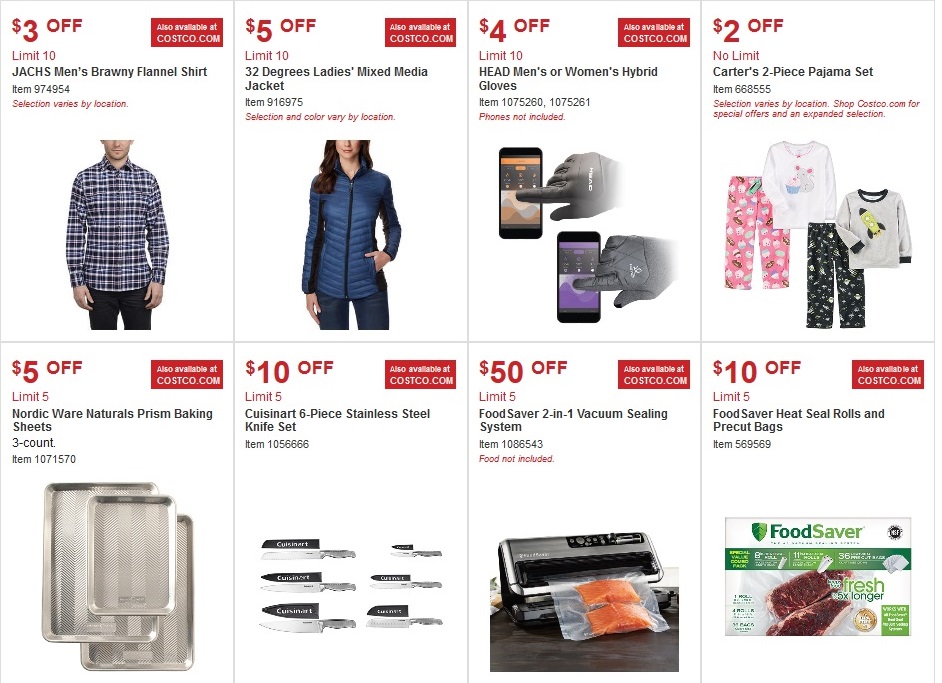This image is a screenshot set against a white background, depicting a page from a shopping website. The layout features eight product listings, organized into two rows of four images each.

In the first row, we observe the following items from left to right:
1. The upper left corner showcases a "Jack's Men's Brawny Flannel Shirt," highlighted with a $3 off discount in bold red text. A red button below states that it is also available at Costco.com, with a purchase limit of 10 per order. The item's identification number is 974954, noted in red. Additionally, there's a disclaimer that selection varies by location. The part-visible image of a man wearing the plaid flannel shirt and dark pants shows him from his nose down to the top of his legs.
2. The next item to the right is a "32 Degrees Ladies' Mixed-Media Jacket," presented with a $5 off discount in red text on a blue jacket.
3. Following this, there's an image of a "Men or Women's Hybrid Gloves."
4. Finally, on the far right of the top row, there is a "Carter's Two-Piece Pajama Set."

In the bottom row, from left to right:
1. The lower left corner presents "Nordic Ware Natural Prism Baking Sheets," illustrated by a photograph of three different-sized silver (aluminum) baking sheets.
2. The remaining products in the bottom row are not described in the provided text.

Overall, this detailed caption provides a comprehensive view of the products and their respective discounts available on the shopping website shown in the image.